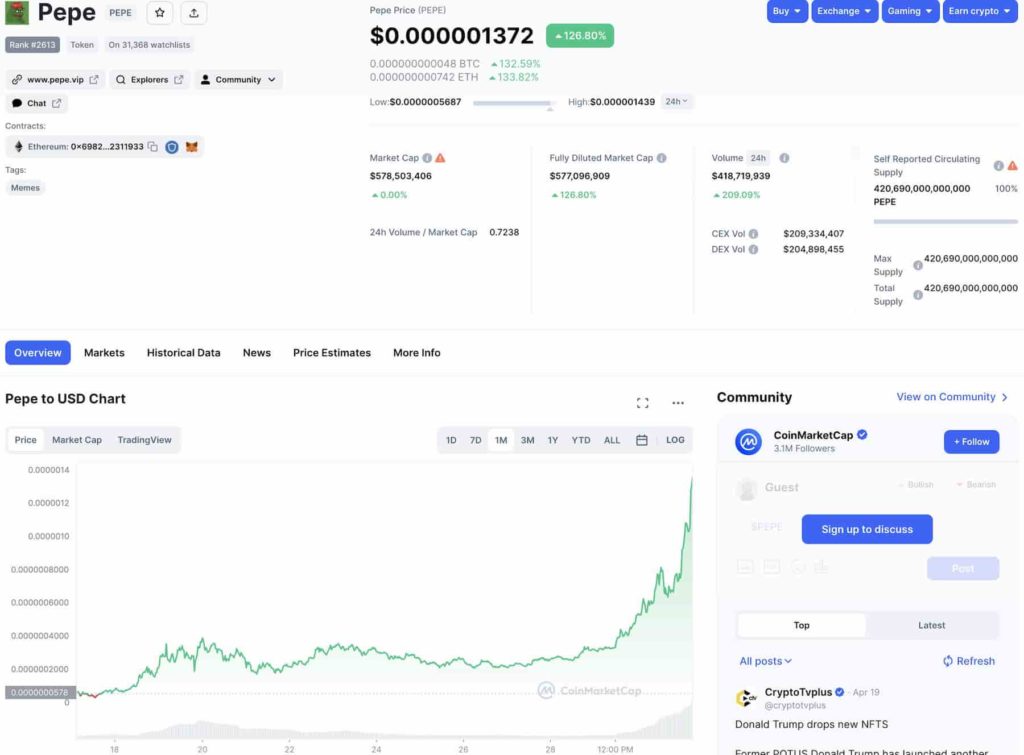Screenshot of a webpage showcasing the PEPE cryptocurrency. In the upper left corner, the website's name "PEPE" is prominently displayed, spelled out as P-E-P-E. Directly below, it mentions that PEPE is ranked number 2613 and is on 31,368 watch lists. Below this, additional details are provided: "pepe.com.vip," along with navigational options such as "Explore," "Community," and "Chat." The associated Ethereum address, "0x69822311933," is also listed, along with the tag "memes."

On the right side of the page, the current price of PEPE is displayed as $0.00001372, indicating a substantial increase of 126.8%. Adjacent to this information, there are interactive buttons for "Buy," "Exchange," "Gaming," and "Earn Crypto," each featuring dropdown menus.

At the bottom of the screen, a chart illustrates the historical performance of PEPE, titled "Pepe USA chart." The chart shows a significant initial low value, marked at approximately 0.000000578, followed by a dramatic increase over time.